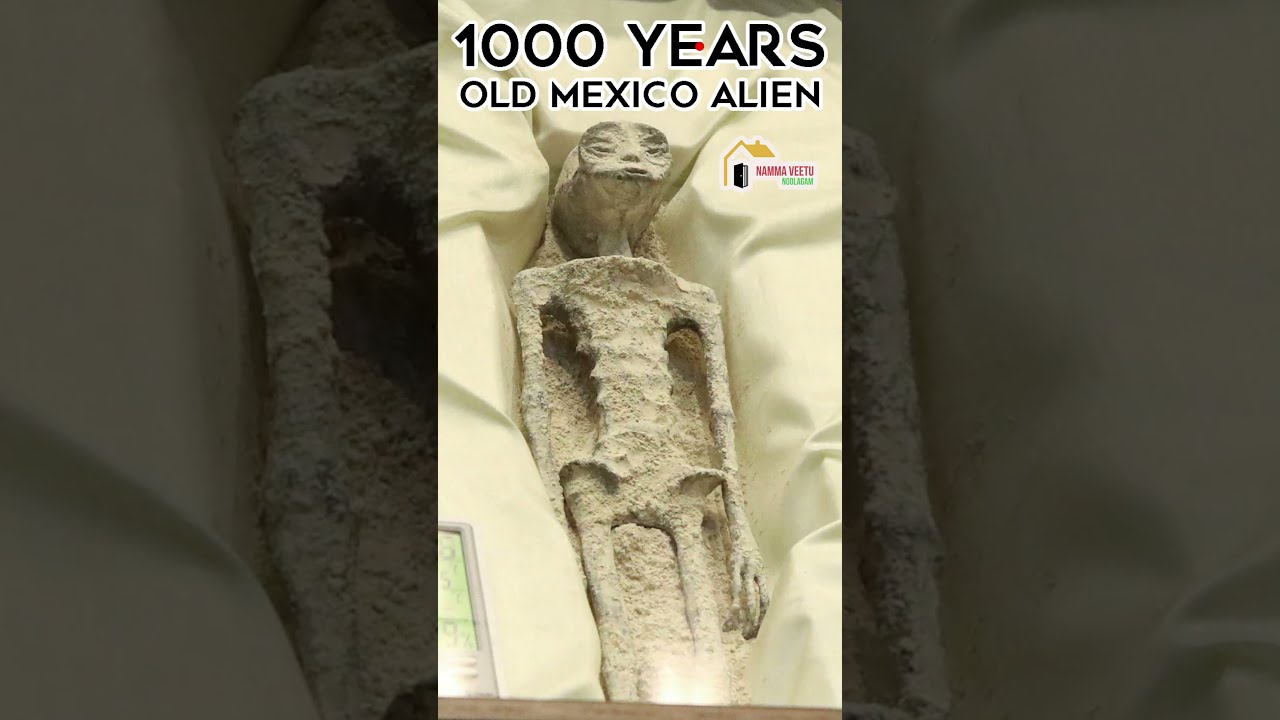The image features an ancient, fossil-like alien skeleton labeled as "1,000-year-old Mexican alien" at the top. The alien figure has a flat, rectangular-shaped head with a rounded back, exhibiting distinct facial features like eyes, a nose, and a small mouth. The skeletal body, appearing to be petrified or made of stone, has thin arms ending in three claw-like fingers, a slender torso, and delicate legs. It is shown laying down on a white or beige sheet that slightly recesses around its body, with some soil visible around it. The backdrop contains various colors and tiny icons, including a house and other indecipherable text. The photo centralizes on the alien figure, unclear if taken indoors or outdoors, and displays a range of colors including dark blue, black, white outlines, red, fuchsia, green, orange, and sandy beige.